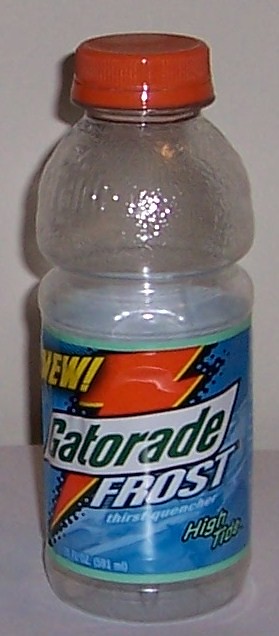A detailed photograph captures an empty Gatorade Frost bottle as the central focus of the image. Prominently displayed above the iconic Gatorade logo, the word "New" heralds this variant. The Gatorade logo itself is a striking orange, providing a sharp contrast against the predominantly blue label. Positioned at the bottom right of the bottle's label, the flavor "High Tide" is clearly indicated along with the capacity, which reads "591 milliliters." The bottle is transparent, allowing a full view of its emptiness, and it features an orange screw-on lid. The text on the label is a mix of yellow, dark green, and white, all presented in a sleek sans-serif font. The photograph appears to have been taken indoors, and a distinct shadow of the bottle is cast on the clean white wall backdrop, giving the image a subtle depth.